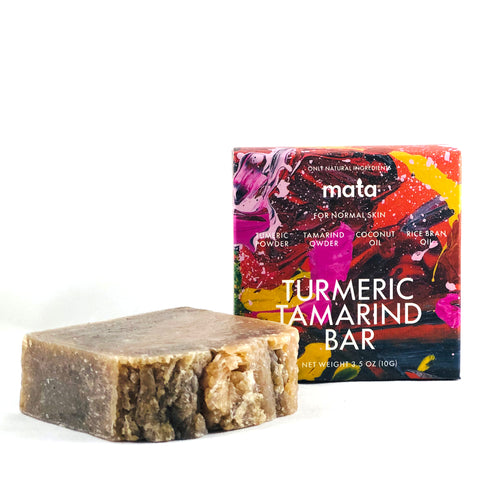The image depicts a bar of soap and its vibrant packaging against a plain white background. On the right side, there is a square package approximately 1.25 inches in both height and width, featuring the word "MATA" at the top center in white print. Below the brand name, it reads "for normal skin", followed by the ingredients: turmeric powder, tamarind powder, coconut oil, and rice bean oil. At the bottom of the package, "turmeric tamarind bar" is written in large white print along with the net weight of 3.5 ounces. The highly colorful packaging includes a mix of pinks, oranges, yellows, reds, and blacks, forming a variety of stripes without a particular pattern. To the left of the package, the actual bar of soap is displayed. It has smooth top, sides, and bottom surfaces, with one edge appearing rough, reminiscent of a broken piece of wood. The soap bar itself exhibits shades of light brown and tan, offering a glimpse of its natural ingredients.